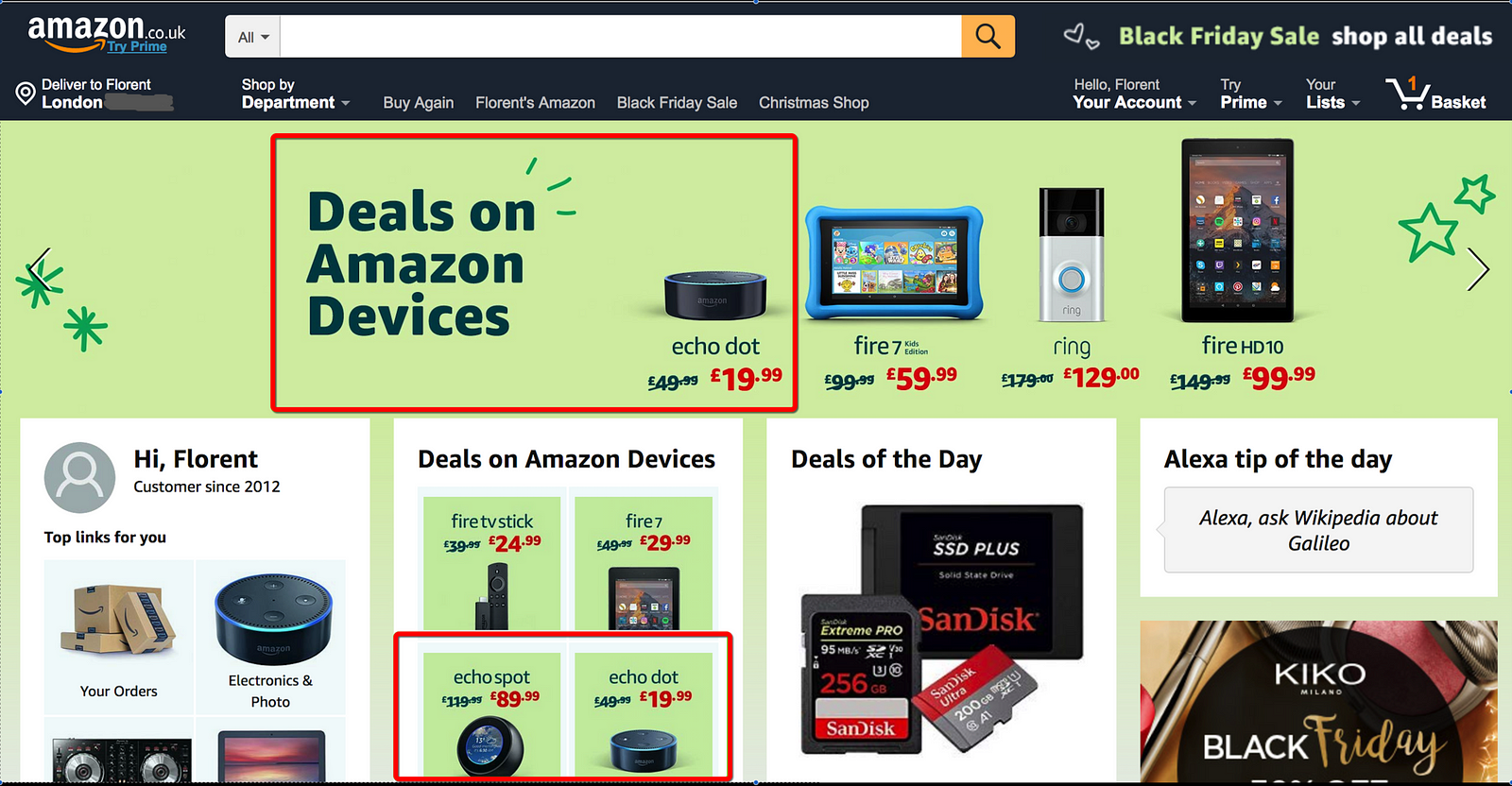Screenshot of Amazon.co.uk Webpage during Black Friday Sales

**Top Navigation Bar:**
- The webpage displays the top navigation bar indicating it is from Amazon.co.uk. 
- On the far left, the Amazon logo is visible.
- To the right, an empty search bar with an "All" dropdown selection is present, accompanied by a magnifying glass icon.
- Adjacent to the search bar, a white banner reads: "Black Friday Sales", and "Shop All Deals."

**Header Section:**
- Below the navigation bar, the header includes options such as "Deliver to Florent, London", "Shop by Department", "Buy Again", "Florent’s Amazon", "Black Friday Sale", and "Christmas Shop."
- The right corner of the header states: "Hello, Florent," with links to "Your Account", "Try Prime", "Your Lists", and an icon of a shopping cart with an orange marker indicating one item in the "Basket."

**Main Page Content:**
- The main content highlights exclusive deals on Amazon devices:
  - **Echo Dot:** Regularly priced at £49.99, now slashed to £19.99 in red text.
  - **Fire Tablet:** Various models of Fire tablets are featured.
  - **Ring Doorbell:** Included among the highlighted Amazon devices.
- The bottom left section welcomes the user: "Hi Florent, Customer since 2012."
  - Below this, personalized recommendations such as "Top links for you:", with options including "Your Orders", "Electronics", and "Photo."

**Additional Offers:**
- Further down, the page outlines:
  - "Deals on Amazon Devices"
  - "Deals of the Day"
  - "Alexa Tip of the Day"

This detailed depiction captures the Amazon.co.uk webpage interface during the Black Friday sales event, highlighting specific deals and personalized touches for the user Florent.